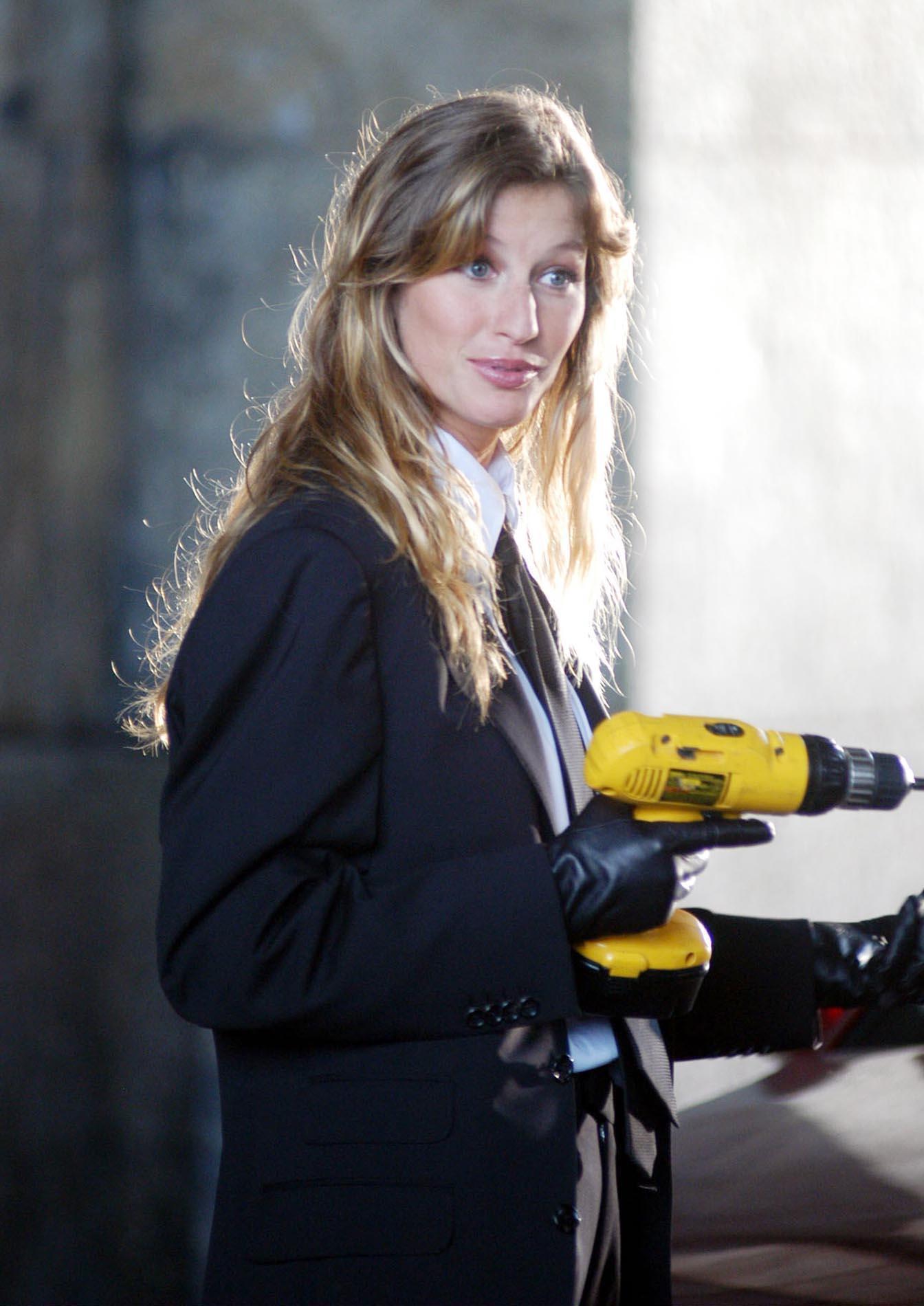The photograph captures a blonde woman with long, slightly wavy hair, standing upright while holding a yellow power drill with a black tip in her right hand. She appears surprised, with wide eyes, and is attired in a navy blue coat over a white collared shirt, paired with black leather gloves. Her attire also features a long black tie. The left half of the image is shadowed, contrasting with the well-lit right half. The background is blurred and predominantly black and white, with the entire image being in color and illuminated by natural light. The scene focuses solely on the woman, highlighting the detailed textures and colors of her clothing and the power drill.